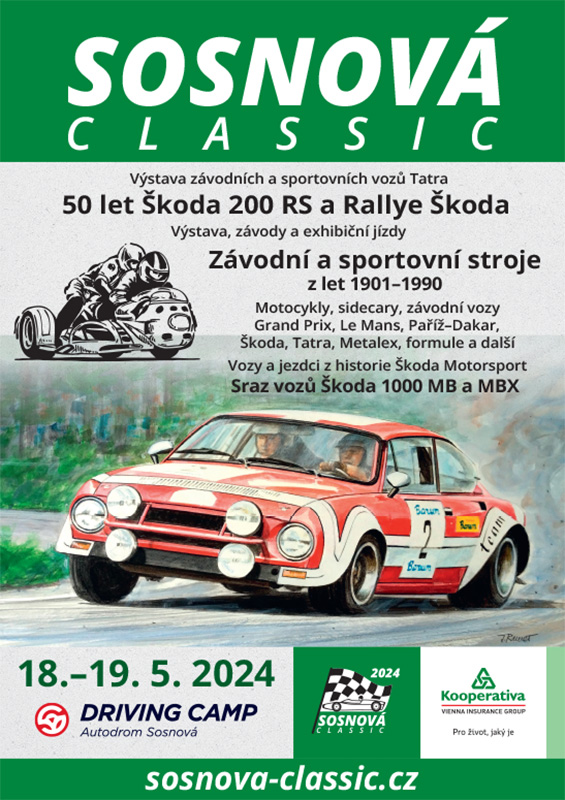The image is a detailed advertisement flyer for the Sosnova Classic 2024 car racing event, set outdoors. It prominently features a top green banner with white text reading "Sosnova Classic." Below this is a gray section with additional details in Czech about the event. Key text includes "Výstava závodních a sportovních strojů z let 1901 až 1990" which translates to "Exhibition of racing and sports machines from 1901 to 1990," mentioning prominent events like Grand Prix, Le Mans, and Paris-Dakar. 

To the left, there's a black-and-white drawing of a motorcycle with two riders, and below this, there’s a striking photograph of a red sports car with the number 2, driven by two men. The central and most eye-catching part of the flyer shows this red car in action, evoking the thrill of racing. Surrounding the car are green grassy areas contrasting with the gray racetrack pavement.

At the bottom, text in green and white includes important details such as the event dates "18-19.5.2024," and venue "Driving Camp, Autodrome Sosnova." A black and white checkered flag is also visible on the right side of the flyer, symbolizing the racing theme. Further down, it mentions sponsors like "Cooperative Vienna Insurance Group," and the event's website, "sosnovaclassic.cz."